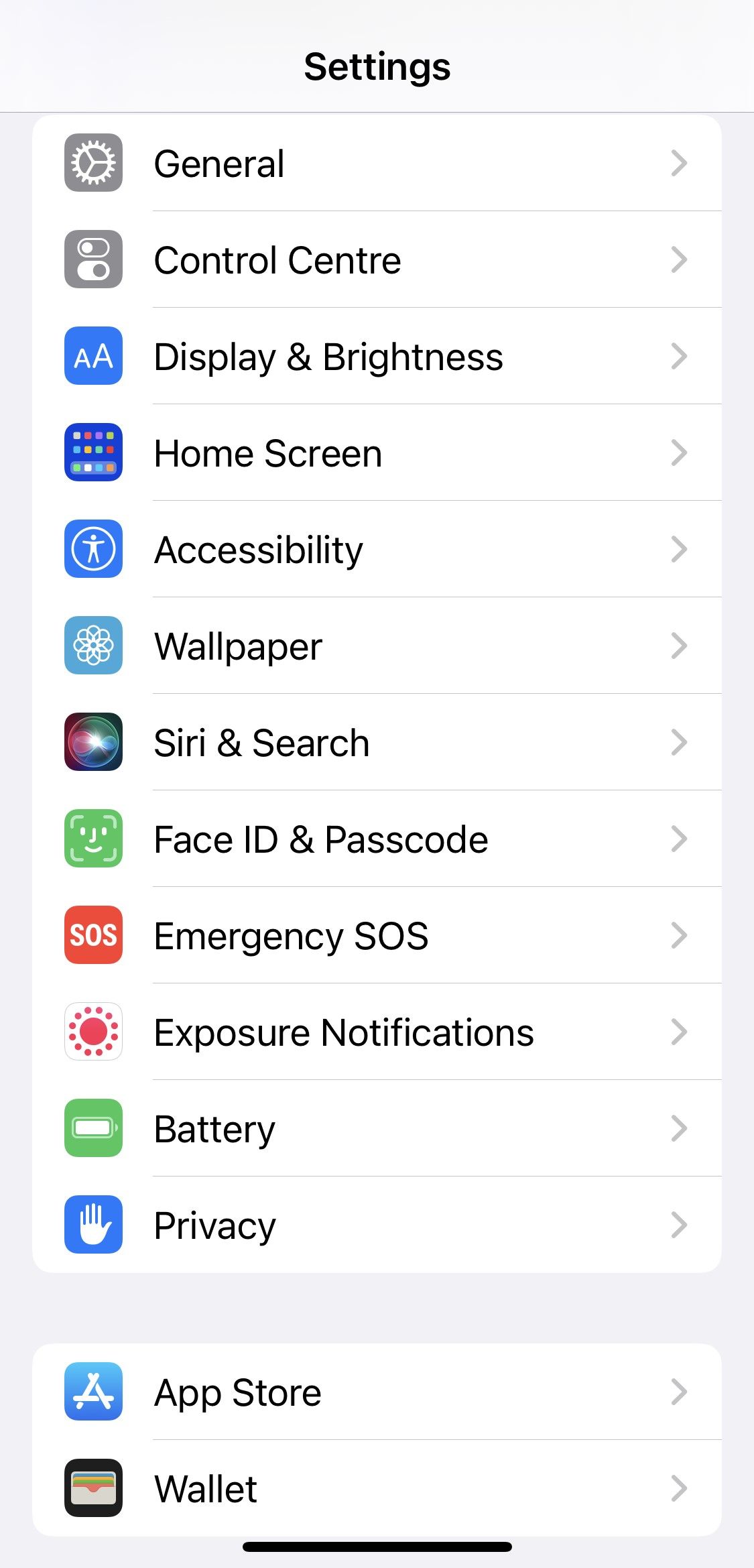The image depicts the Settings page of an iOS operating system on a mobile device, which could be either an iPad or an iPhone. The main screen displays a comprehensive list of various categories and apps included with the operating system. Each category is aligned with a corresponding icon on the left and features an expansion arrow for accessing additional menus.

The visible categories in this screenshot include:
1. General
2. Control Centre (indicating UK English settings)
3. Display & Brightness
4. Home Screen
5. Accessibility
6. Wallpaper
7. Siri & Search
8. Face ID & Passcode
9. Emergency SOS
10. Exposure Notifications
11. Battery
12. Privacy

Below these categories, in a separate section, two additional options are visible:
1. App Store
2. Wallet

The page layout is typical for iOS settings, combining intuitive navigation with iconography for ease of use. The British spelling of 'Centre' in 'Control Centre' suggests that the device is set to UK English.